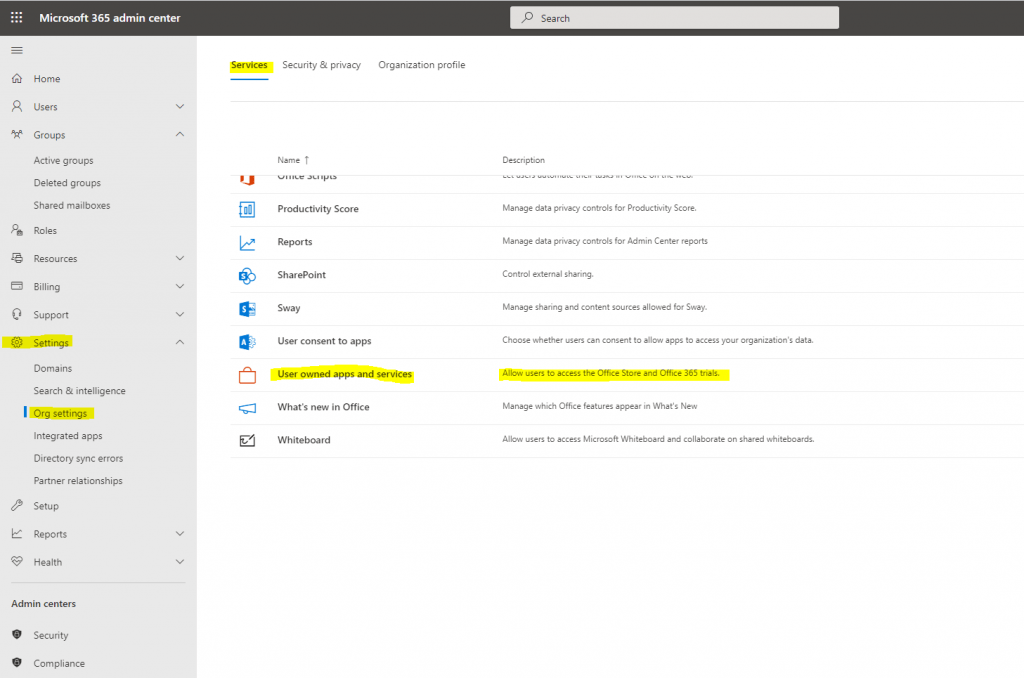This image is a digital screenshot of the Microsoft 365 Admin Center, focusing on the 'Services' tab, which is highlighted. Detailed options and descriptions visible include:

1. **Productivity Score**: Manage data privacy controls for the productivity score.
2. **Reports**: Manage data privacy controls for admin center reports.
3. **SharePoint**: Control external sharing settings.
4. **Sway**: Manage sharing permissions and content sources allowed for Sway.
5. **User Consent to Apps**: Decide whether users can consent to allow apps to access your organization's data.
6. **Use Your Own Apps and Services**: This section is highlighted, including its description, which outlines that it allows users to access the Office Store and Office 365 trials.
7. **What's New in Office**: Manage which Office features appear in the 'What's New' section.
8. **Whiteboard**: Allow users to access Microsoft Whiteboard and collaborate on shared whiteboards.

The 'Use Your Own Apps and Services' option and its description are both highlighted, indicating a particular focus or attention within the interface.